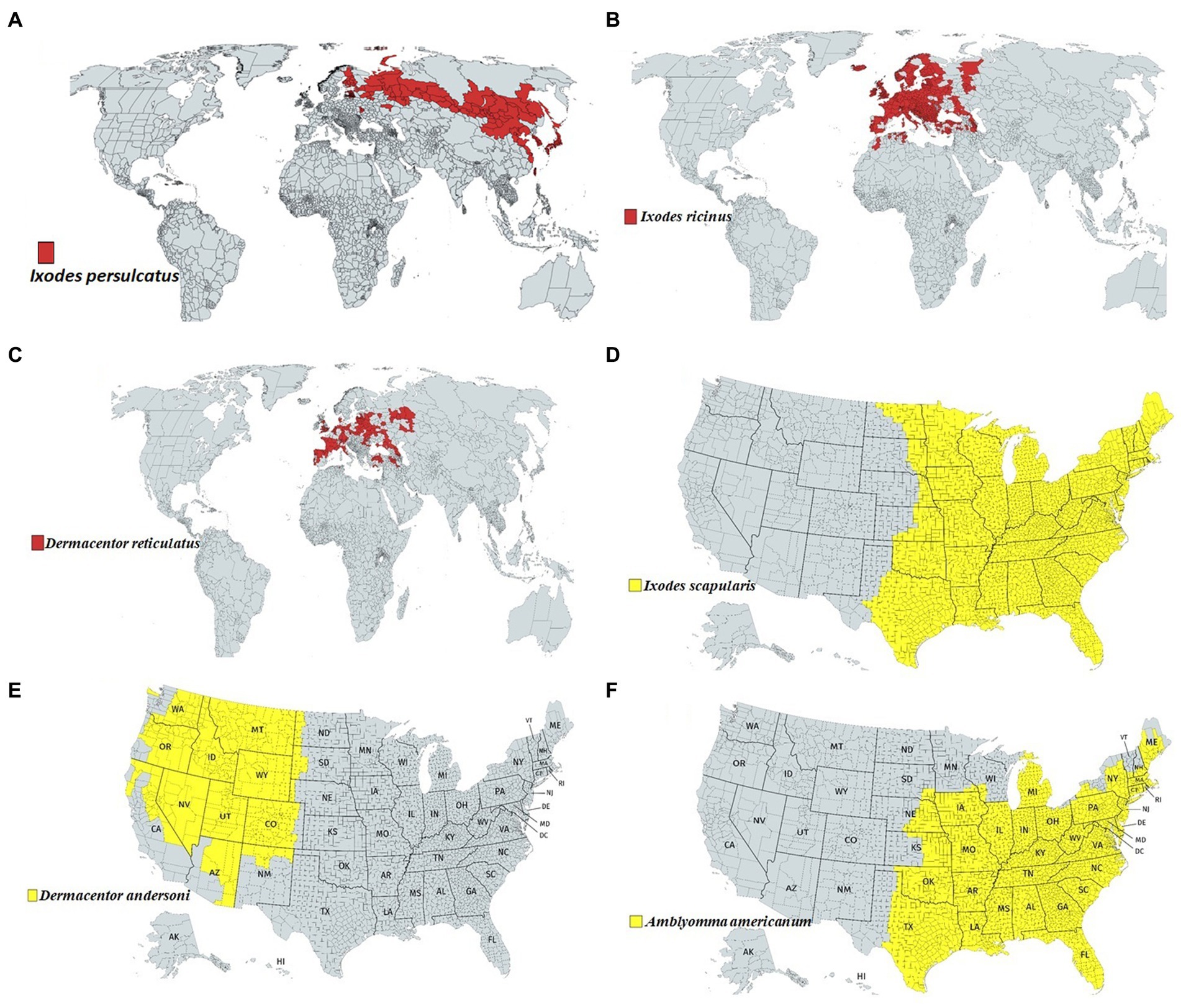The image features six maps, categorized as three world maps and three United States maps, each indicating various geographical regions in specific colors. The world maps, labeled A, B, and C, display regions in shades of gray with certain areas highlighted in red. Map A, titled Ixodes Persulicatus, highlights parts of Europe, particularly around Russia and China. Map B, labeled Ixodes Ricinus, covers much of Europe, parts of Northern Africa, and regions near Russia and China. Map C, titled Dermacentor Reticulatus, shows scattered red zones mainly in central Europe. 

The U.S. maps, labeled D, E, and F, are in shades of gray and yellow. Map D, indicated as Ixodes Scapularis, shows the eastern half of the U.S. in yellow, including states like Texas, Oklahoma, Kansas, and Nebraska. Map E, titled Dermacentor Andersoni, highlights western states such as Washington, Oregon, Colorado, Montana, and parts of California and Arizona. Map F, labeled Amblyomma Americanum, primarily covers the southeastern U.S. in yellow, including parts of Texas, Oklahoma, Kansas, and certain northeastern states like New York and Maine. 

These maps are arranged in two columns: to the right, there is a world map on the top, a U.S. map in the middle, and another U.S. map at the bottom; to the left, a world map atop, followed by another world map, and ending with a U.S. map. Each map is accompanied by a colored rectangle providing contextual titles and labels, although the text is in a foreign language.